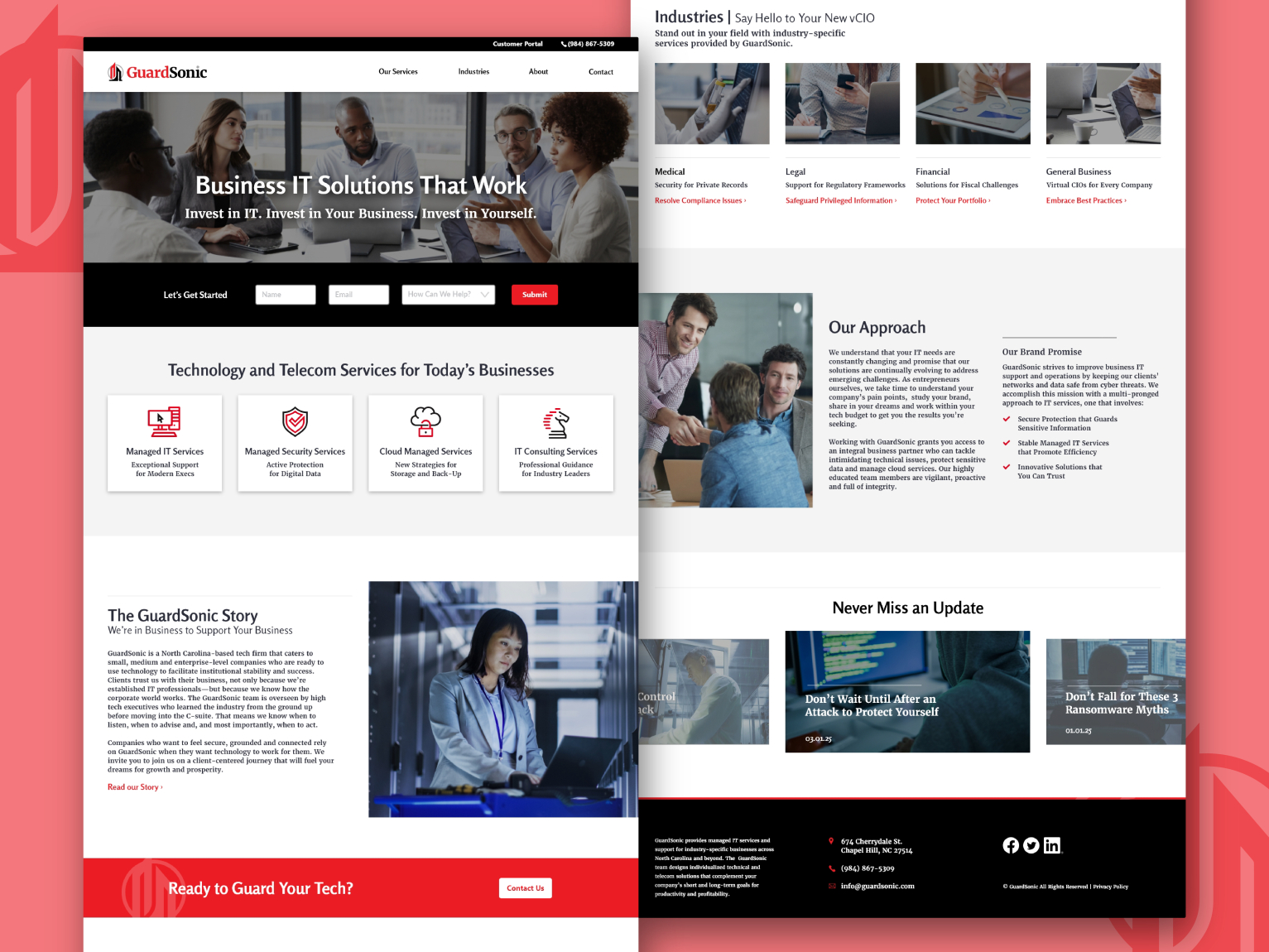The caption should read:

"This image showcases a detailed visual representation of a website designed for viewing on a tablet, such as an iPad. In the top left corner of the primary image, the brand name 'Guard Sonic' is prominently displayed. In the top right corner of the screen, some text is visible but difficult to read. Beneath this section, there is a large image depicting a professional meeting. Overlaying this image are the words: 'Business IT Solutions That Work. Invest in IT, Invest in Your Business, Invest in Yourself.' Below this, a call-to-action button that reads 'Let's Get Started' is positioned alongside input fields presumably meant for entering your company name or your personal name, next to a red 'Continue' button.

Following this, the website mentions, 'Technology and Telecom Services for Today's Business,' accompanied by several icons. The first box below this section indicates 'Managed IT Services,' followed by 'Managed Security System Services,' 'Client Managerial Services,' and 'IT Consulting Services.' 

Further down, there is a segment titled 'The Guardian Story,' featuring an image of a woman working on a computer. On the right-hand side of the display are four images arranged at the top, with a picture of three individuals in a meeting beneath the heading 'Our Approach.' Below this, another section reads 'Never Miss an Update,' accompanied by three additional images. The webpage concludes with a black bar displaying standard company information, including location, phone number, and address."